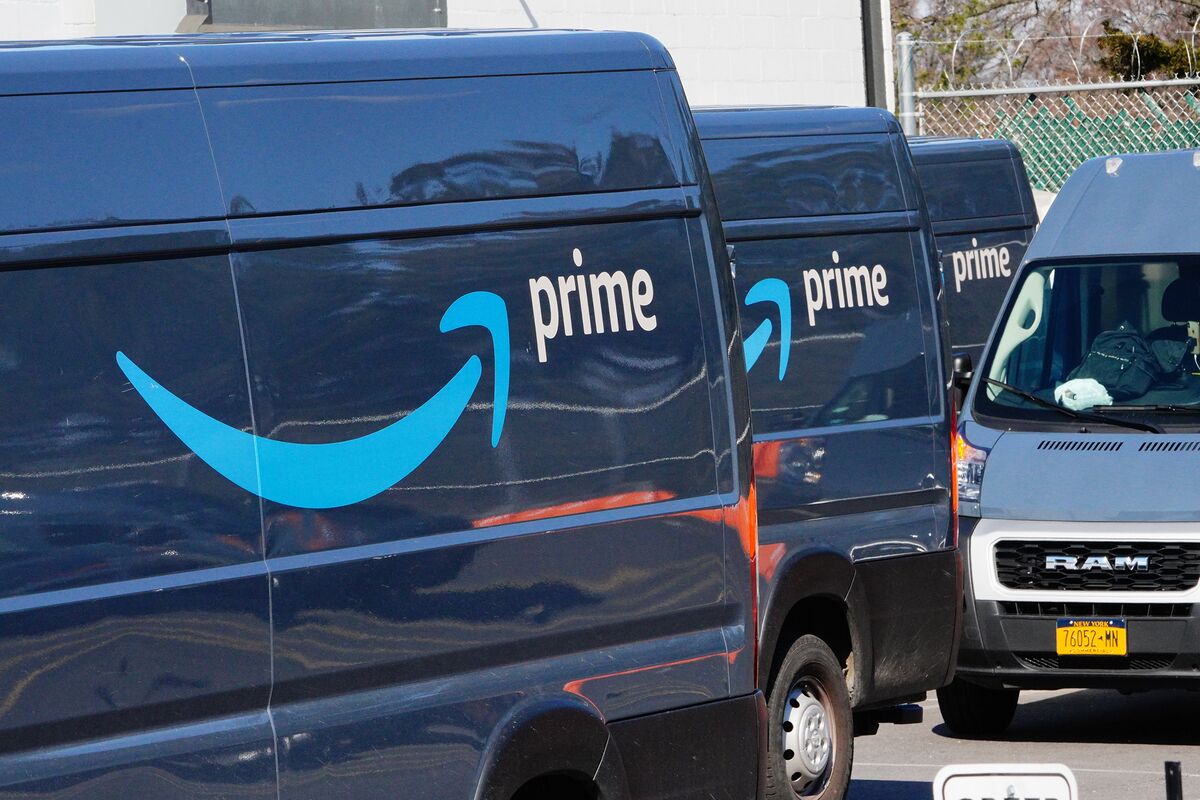In this vibrant outdoor image, several Amazon Prime delivery trucks are prominently featured. The scene appears to be set in a parking lot adjacent to an Amazon facility, accentuated by a clear, sunny sky. At the top right, a high fence with barbed wire underscores the secure nature of the location. The focus of the image is on the fleet of Amazon Prime delivery vehicles—dark blue box vans with the distinctive Prime logo displayed on the rear. At least three of these blue vans are visible, suggesting a day of bustling activity ahead. Additionally, a gray minivan, branded with the "Ram" logo, is parked among the Amazon trucks, raising questions about whether it is part of the fleet or simply a coincidental presence. The overall bright and sunny atmosphere highlights the vivid colors and details of the vehicles and surroundings.